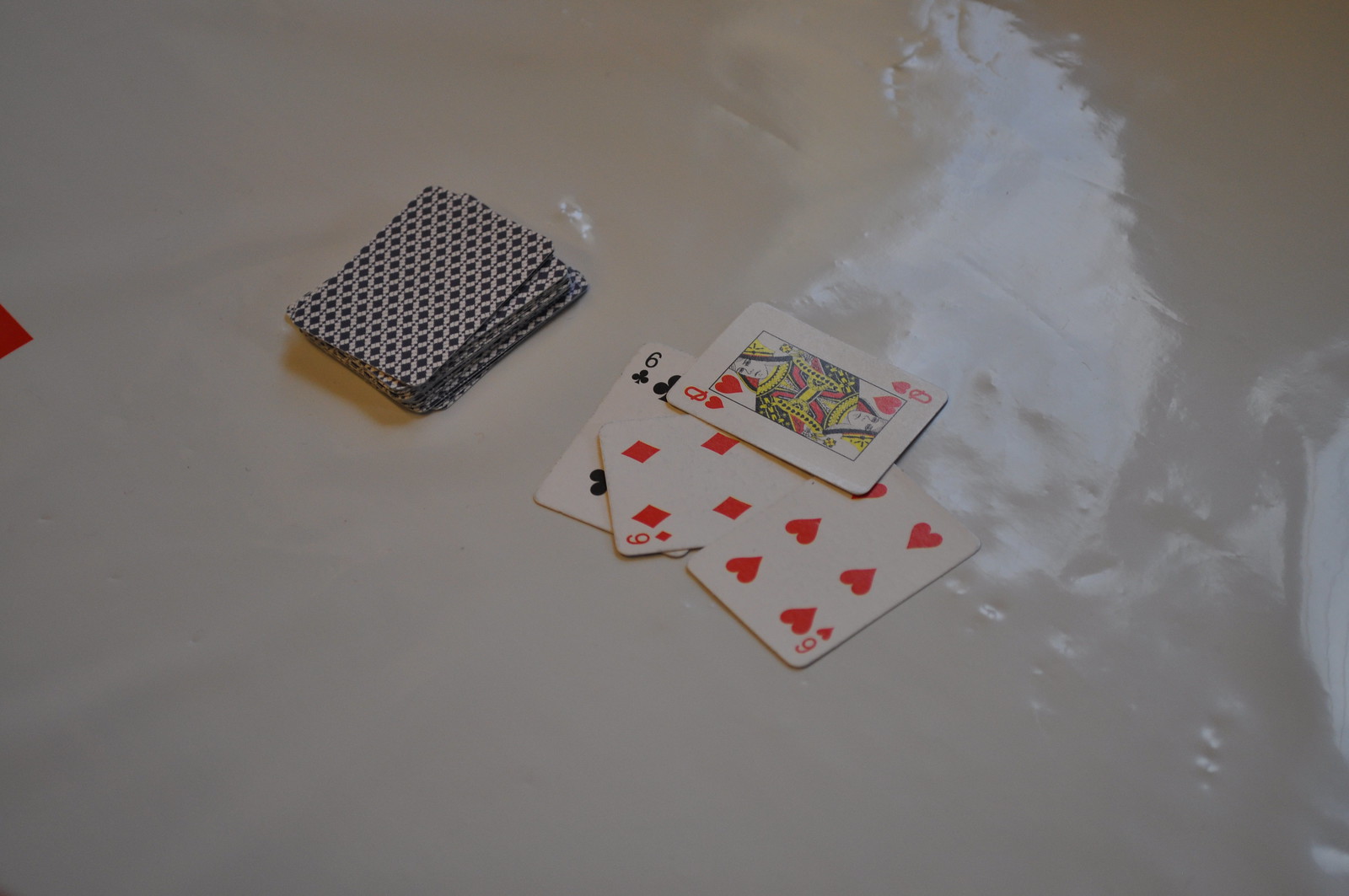This photograph, taken in low light, captures a deck of cards predominantly face down, showcasing their intricate navy blue and white diamond-patterned backs. To the right side of the image, four cards are loosely stacked in varying orientations. The bottom card is a black Six of Clubs, followed by a red Six of Diamonds, a red Six of Hearts, and finally, a red Queen of Hearts. In the far left corner, there is an ambiguous red object, possibly a piece of paper, partially visible. The light source reflects off the upper right corner of the face-up cards, highlighting the texture of the plastic sheeting or tabletop cover on which they rest. The plastic surface has several small punctures, adding to the overall detail of the scene.